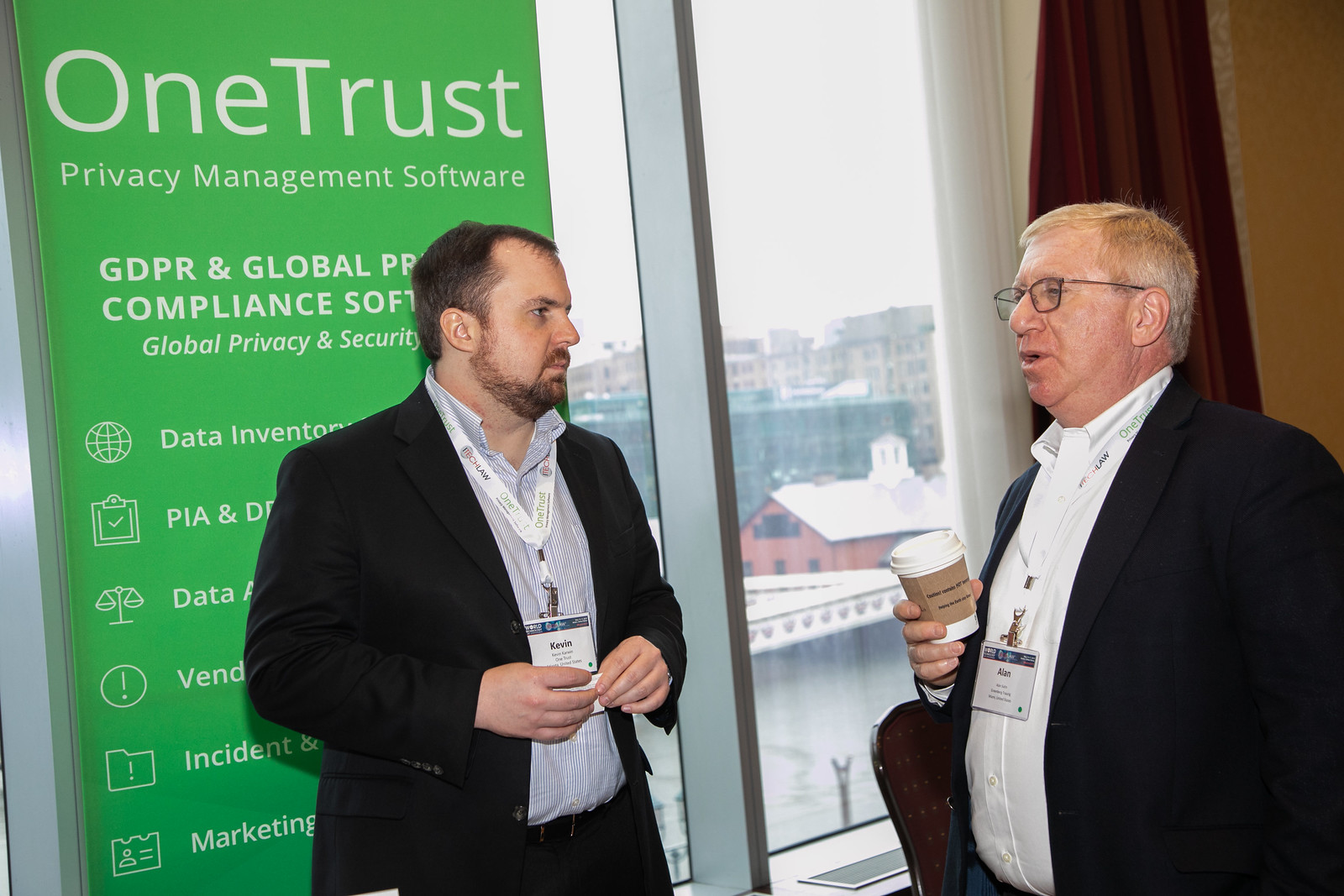In the photo, two men are engaged in conversation near a large window with a view of a cityscape. The man on the left has short brown hair, a light beard, and a receding hairline. He is dressed in a suit jacket and an unbuttoned collared shirt, and wears a white name tag on a lanyard around his neck, which reads "Kevin." His hands are clasped in front of his chest. Behind him is a green poster displaying white text, partially obscured by his head, that reads "OneTrust Privacy Management Software" and "Global Privacy and Security." The text suggests features the software offers, such as Data Inventory, PIA, and Marketing, although some words are covered.

The man on the right appears older, possibly in his late 50s or 60s, with fair hair and glasses. He is also wearing a suit jacket with a white button-down shirt, and has a similar name tag which reads "Alan." He holds a small coffee cup with a brown cardboard sleeve and seems to be speaking. The setting appears to be a convention or conference, indicated by the professional attire and informational poster. A red curtain hangs to the right of the window.